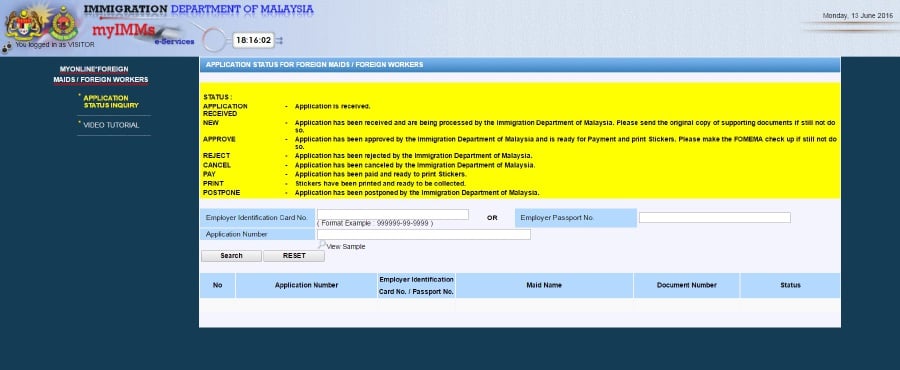This image is a screenshot displaying an informational webpage from the Immigration Department of Malaysia. The background features a prominent blue banner running horizontally from left to right. In this banner, the word "Immigration" appears in bold black text, while "Department of Malaysia" is written in blue text. Below this banner, in red text, it reads "my MMS eServices".

Underneath is a notification stating, "You logged in as a visitor." Below this message is a yellow box with a blue header that indicates the "Application Status for Foreign Maids and Foreign Workers." The current status displayed is "Application Received," with the message, "New application has been received and is being processed by the Immigration Department of Malaysia. Please send the original copy of supporting documents."

Further down the page, various possible application outcomes are listed:
- "Application has been approved" by the Immigration Department of Malaysia.
- "Application has been rejected" by the Immigration Department of Malaysia.
- "Application has been cancelled" by the Immigration Department of Malaysia.
- "Application has been paid and ready to print stickers."
- "Stickers have been printed and ready to be collected."